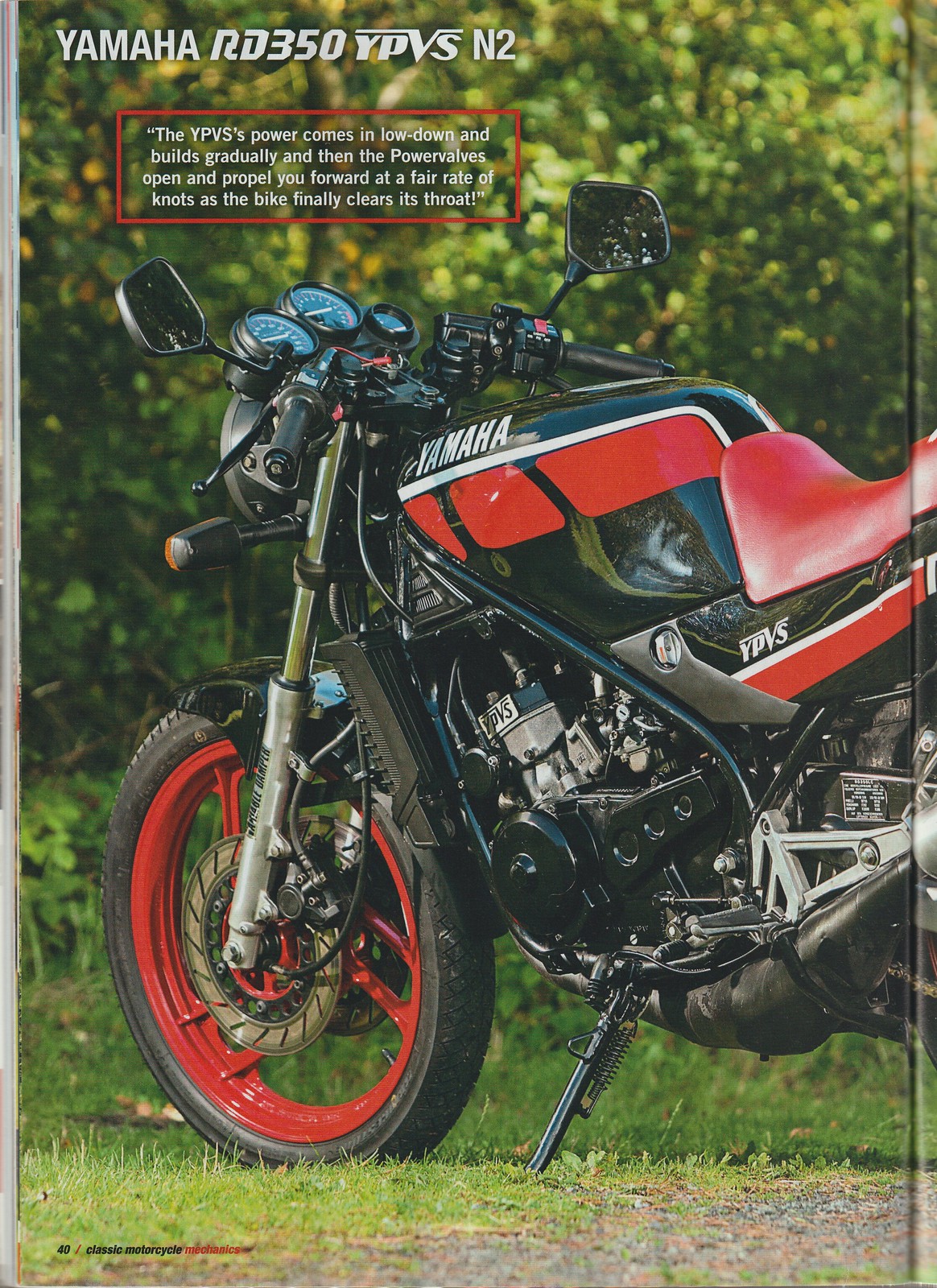The image is a scanned page from an auto magazine, featuring the iconic Yamaha RD350 YPVS N2 motorcycle. Positioned at the center-left of the portrait-oriented page, the motorcycle is angled to the left, its front half prominently displayed. The bike is parked on a grassy patch with a lush, green, wooded background, creating a vivid and dynamic outdoor setting.

The Yamaha RD350 showcases a striking color scheme with a red seat, black fuel tank adorned with red squares, and a white stripe extending from the front to the seat, proudly displaying the Yamaha logo in bold white capitals. The front wheel features an eye-catching red rim with a black outer tire, connected by a silver bar. Additional details include visible handlebars, tires, and wing mirrors at the top of the image.

A more detailed examination reveals white text at the top left corner of the page that reads "Yamaha RD350 YPVS N2." Below this, a red-bordered text box delivers an evocative description of the bike's performance: "The YPVS's power comes in low down and builds gradually. And then the power valves open and propel you forward at a fair rate of knots as the bike finally clears its throat."

Towards the bottom of the image, more text is visible, including "40 / Classic Motorcycle," albeit some red text remains unreadable. The image, likely part of a two-page spread in a classic motorcycle section, effectively captures the essence and allure of the Yamaha RD350, blending descriptive text and vivid imagery to highlight the bike's design and performance in a picturesque environment.